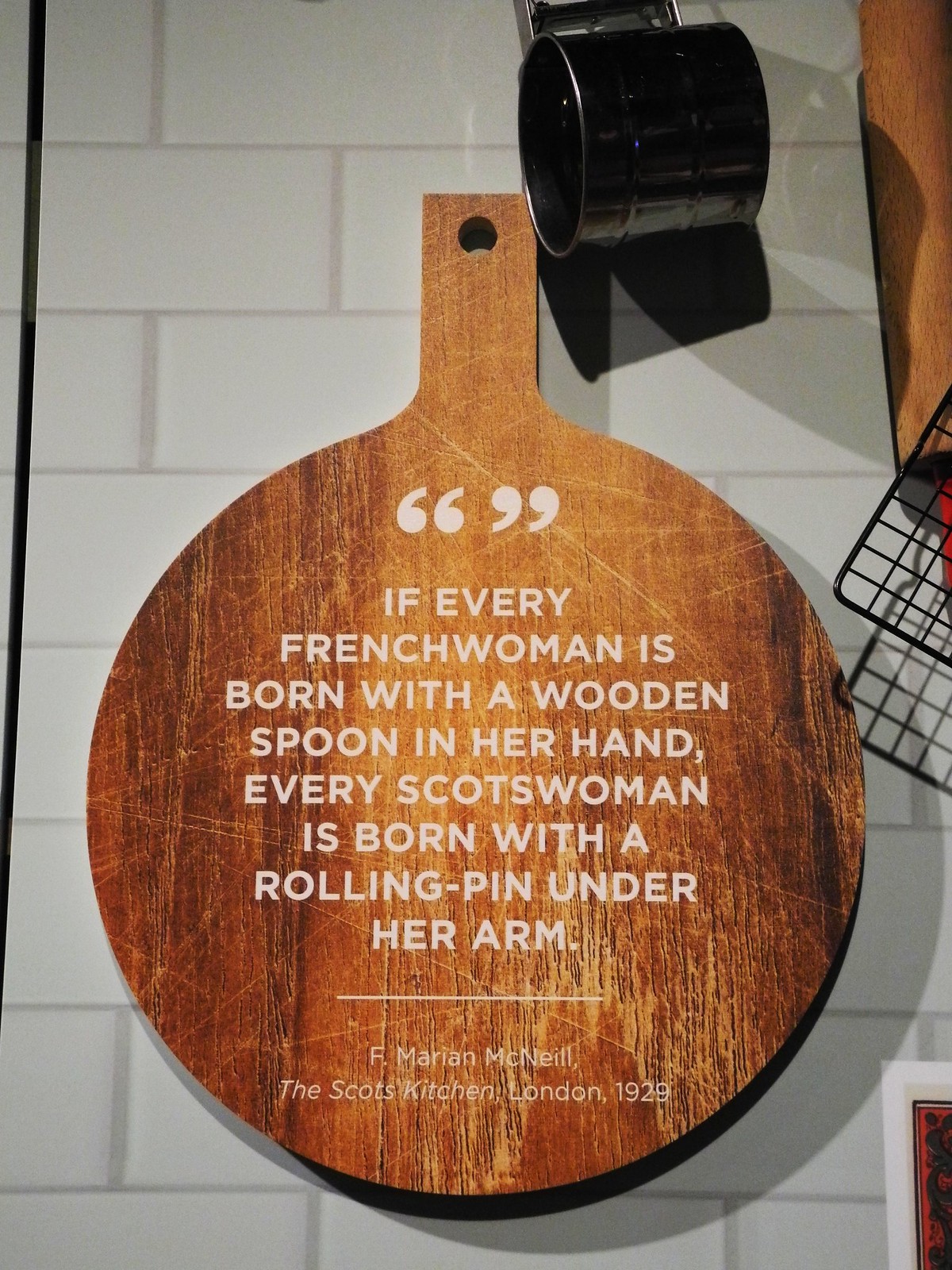This image captures a quaint kitchen scene featuring a well-loved, medium-toned wooden cutting board, adorned with visible cuts and marks that speak to its frequent use. The cutting board, which possibly doubles as a pizza peel, is round in shape and hangs on a white subway tile backsplash. Alongside it, a black mug also hangs from the wall, adding to the rustic kitchen aesthetic.

A charming quote adorns the center of the cutting board, rendered in white text. The quote reads, "If every French woman is born with a wooden spoon in her hand, every Scotswoman is born with a rolling pin under her arm." This phrase is attributed to F. Marion McNeill from her book, "The Scots Kitchen, London, 1929," indicated in smaller white text below the main quote. This thoughtful addition gives the kitchen scene a touch of literary nostalgia and cultural homage.